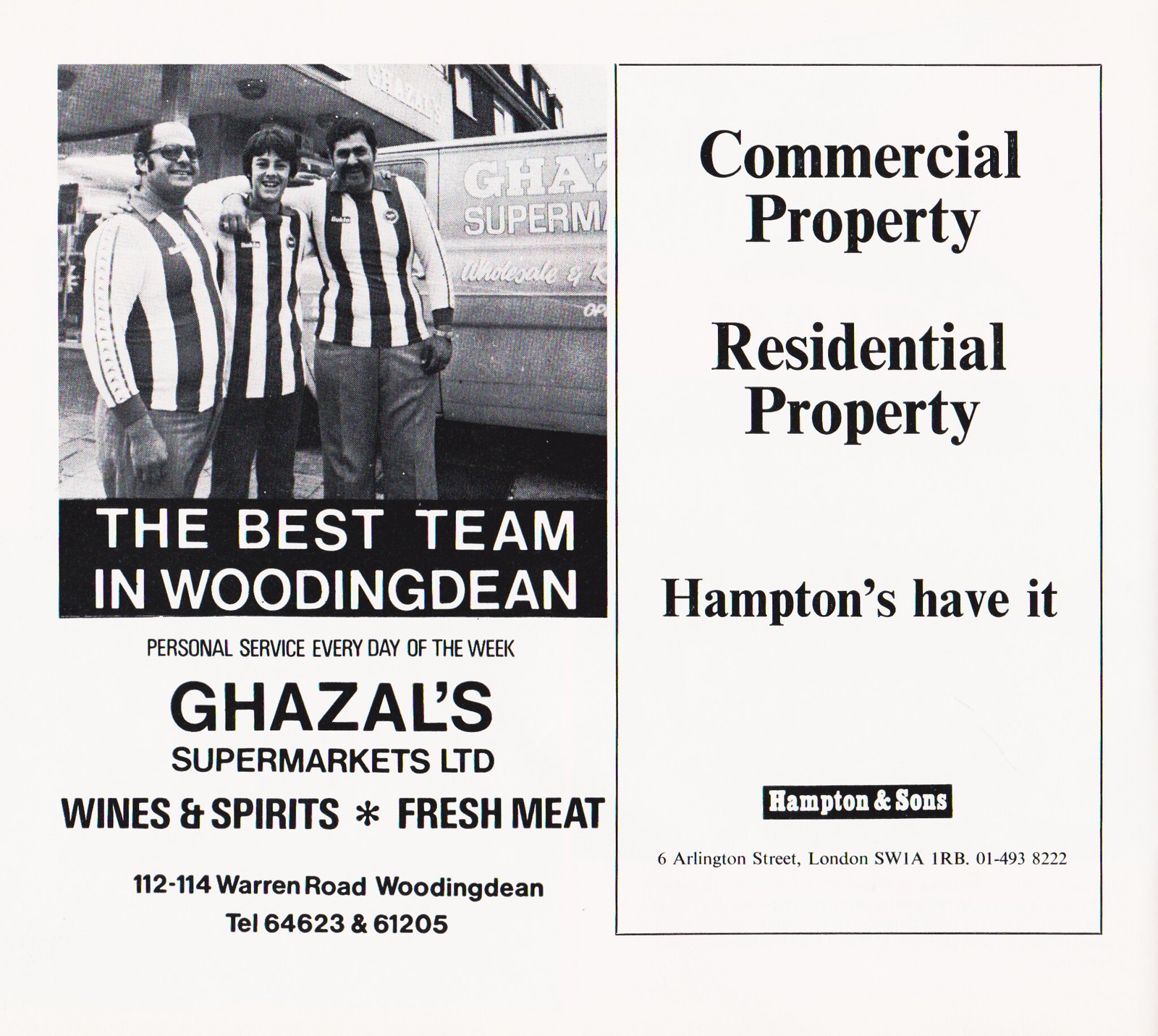This is a detailed black-and-white advertisement flyer printed on an off-white background with black ink. The upper left-hand corner features a black-and-white photograph of three smiling men, each dressed in black-and-white striped, long-sleeved uniforms with dress pants. The men, standing cheerfully beside a van and a building, appear to be of different ages—one in his 20s in the center, flanked by two others who look like they're in their 40s. The man in the center wears sunglasses. Below the photograph, a black band with white text proudly proclaims, "The Best Team in Woodingdean." Following that, it reads, "Personal Service Every Day of the Week." Bold text underneath highlights "Dawesville Supermarket Ltd." offering "Wines and Spirits and Fresh Meat" at "112-114 Warren Road, Woodingdean." To the right of the image, bordered by a black frame, additional bold text details services like "Commercial Property, Residential Property" provided by "Hamptons Havoc, Hampton & Sons," with the business address at the bottom.